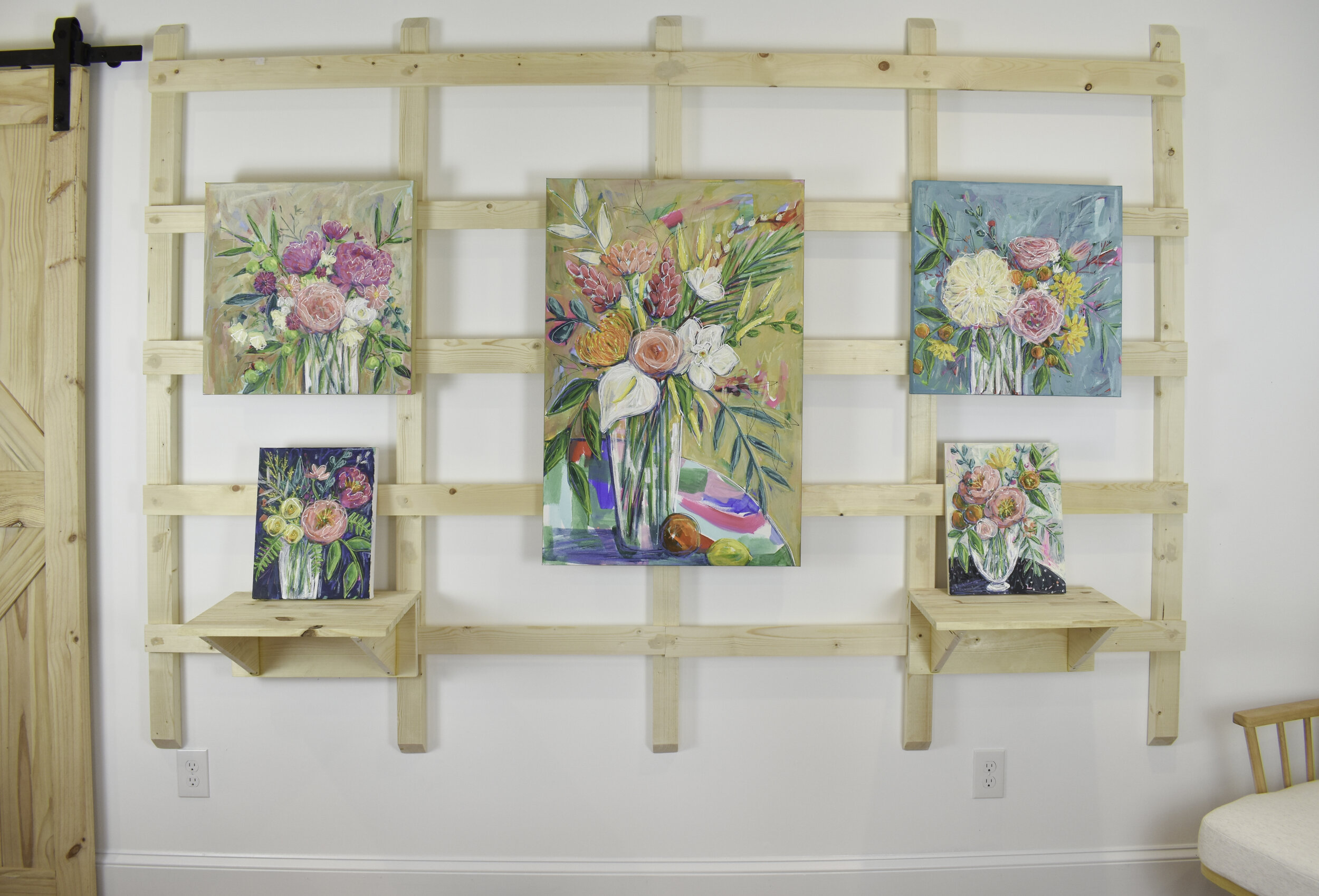The photograph captures a charming room with whitewashed walls, showcasing a series of five paintings mounted on a rustic wooden frame. This wooden frame, made of planks that have been boarded and nailed together, hangs prominently on the wall. Each painting within the frame depicts an array of flowers in vases, rendered in a mix of pastels and vibrant colors, including greens, blues, purples, yellows, reds, and whites. The flowers vary in type and composition, bringing diversity and beauty to the display. On the far left edge of the image, a light wood-colored sliding door with a black hinge is visible, adding a touch of rustic charm. In the lower right corner, part of a wooden chair with a white cushion can be seen, emphasizing the cozy and intimate nature of the space. This elegant arrangement of flower portraits, which appear to be oil paintings, creates a serene and aesthetically pleasing focal point in the room.